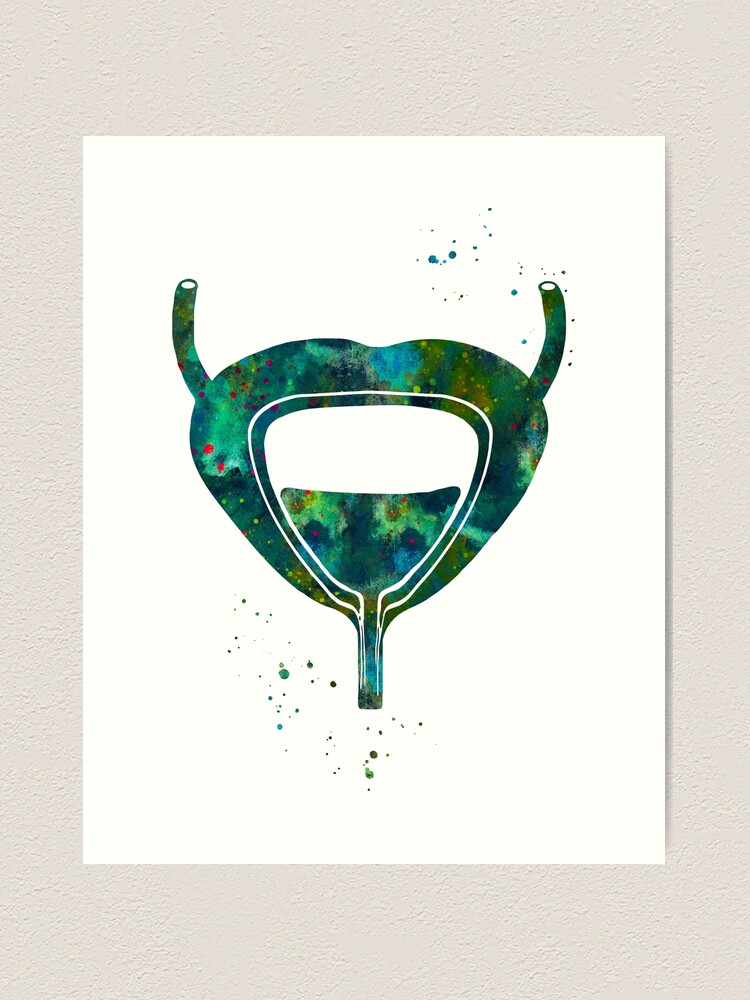This image portrays a vibrant watercolor painting on white paper mounted against a textured beige wall. The central figure in the painting is an abstract, rounded-triangle shape with tube-like appendages protruding from its top corners and bottom point. The shape evokes various interpretations, such as a stylized heart, an alien head, or even a component of a woman's reproductive system.

The painting predominantly features a marbled pattern of blue and green hues, interspersed with red splatters and specks of several colors—green, blue, red, and purple. Within the central shape, there is a distinct white outline that follows its triangular form. Inside this outline, a thin strip of the same marbled pattern frames a rounded rectangle of blank white space at the center. The two upward-pointing tubes end in white circles, suggesting hollow interiors.

Externally, the piece is decorated with additional splatters of green and blue paint, contributing to its dynamic and speckled appearance. The combination of bold, varied colors and the swirling marbled effect gives the piece a galaxy-like, otherworldly aesthetic.